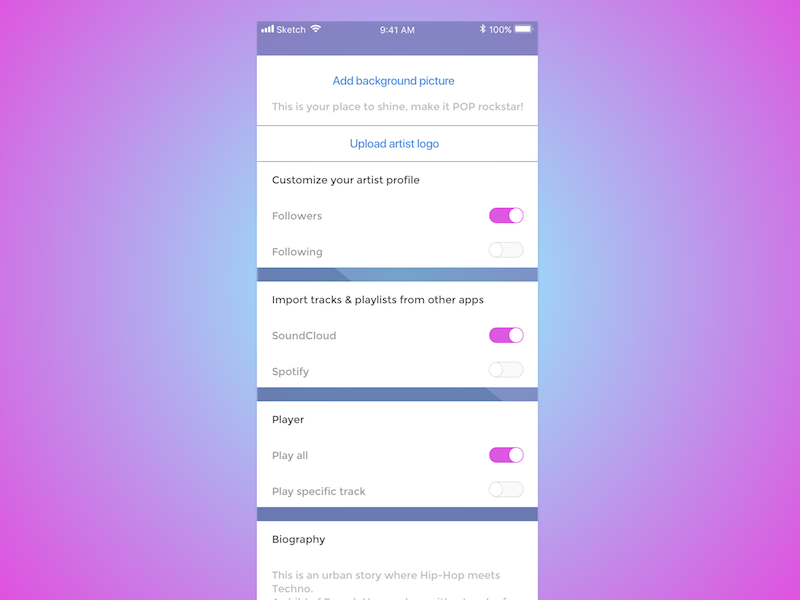This image is a detailed screenshot of a mobile phone interface set against an aesthetically pleasing background. The background features a bluish center with a subtle pink misty outline enveloping the sides, top, and bottom. The upper-left corner of the screenshot displays a full signal strength of five bars. Beside it, an icon of a capital 'S' denotes the app in use, followed by the Wi-Fi signal, indicating that the device is connected to a network. The time is shown at 9:41 a.m., accompanied by a Bluetooth icon and a fully charged battery at 100%.

Below this status bar, the first white panel provides user instructions in a visually engaging manner. In blue text, it prompts: "Add background picture." Beneath this, gray text encourages: "This is your place to shine. Make it pop, rock star!" 

A thin gray line separates this from subsequent navigation options. "Upload artist logo" is highlighted in blue text, followed by another gray dividing line. Below, in black text, it states: "Customize your artist profile," accompanied by toggles for "Followers" and "Following." The "Followers" option is activated, highlighted in pink, with the circle moved to the right, whereas "Following" is inactive, in gray, with the circle positioned left.

Further down, another blue line delineates the next section. The following white panel features "Import tracks and playlists from other apps" in black text. SoundCloud is selected, denoted by a pink circle moved to the right, while Spotify remains unselected, in gray, with its circle to the left.

The succeeding white panel is labeled "Player" in black text. It offers the option to "Play all," which is selected and marked with a pink circle to the right, while "Play specific track" remains unselected, in gray, with its circle to the left.

The final white panel is tagged "Biography" in black text. It begins with the description: "This is an urban story where hip-hop meets techno," but the rest of the text is cut off, leaving an element of mystery.